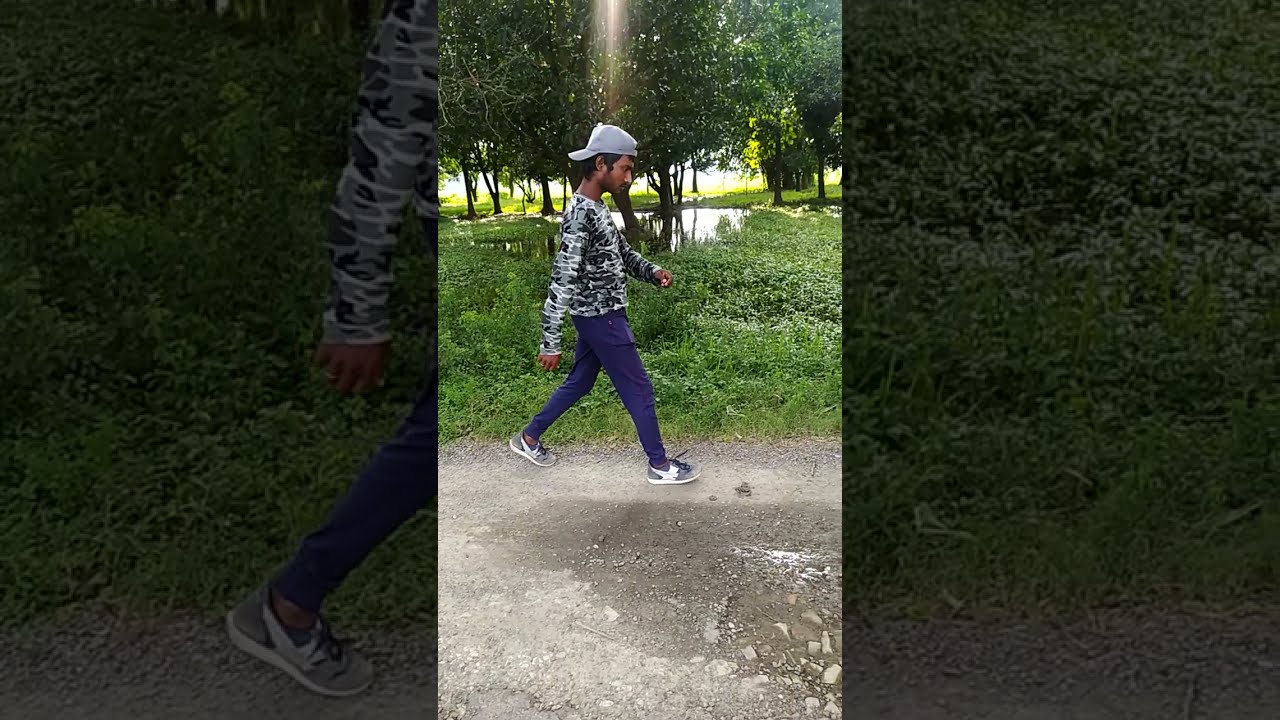The image captures a young man, who appears to be of Middle Eastern descent, walking down a moist, gray dirt path scattered with tiny rocks, situated in a park-like setting. The scene is framed with luscious green trees, including small tree trunks and bushy, leafy foliage, enveloping the pathway. Behind the man, toward his left shoulder, a small pond is visible, adding to the serene atmosphere. The area surrounding the pond features a large grassy plot, intertwined with weeds and reflecting natural sunlight. The man, who has brown skin and black hair, is dressed in a gray baseball cap worn backward, a black, white, and gray camouflage long-sleeve shirt, blue pants that subtly take on a purple hue, and gray and white running shoes. The image, possibly a screenshot from a TikTok or Instagram reel, has an aspect ratio typical of a smartphone capture. The main photo also includes close-up fragments on the left and right sides, detailing parts of the man's arm and leg, as well as the grassy surroundings, further enhancing the scene’s context. Sunlight peeks through the trees, reflecting off the man's hat, enriching the outdoor ambiance.